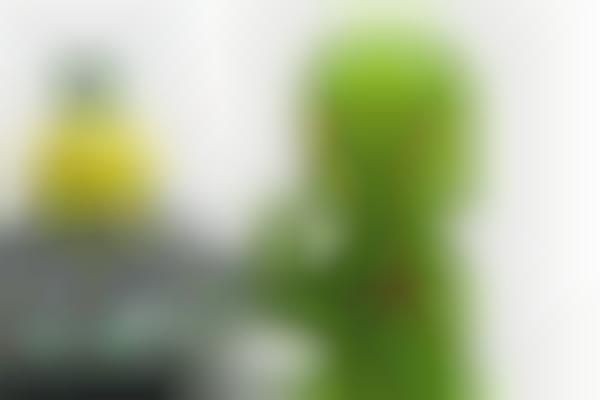The image is very blurry and out of focus, making it difficult to clearly identify the subjects. On the right-hand side, there appears to be a greenish figure with human-like or Muppet-like proportions, possibly resembling Kermit the Frog or an alien. This figure has a bulbous area at the top that could be interpreted as a head, with an appendage that might be an arm. There is a spot of red around the chest area, suggesting a location around the heart, and one arm seems to be bent towards the mouth, potentially indicating the figure is sucking its thumb, leading one viewer to speculate it might be a child. On the left side of the image, there's a grayish blob with a yellow round top that bears a black dot, somewhat resembling Bert from Sesame Street or possibly mimicking a cactus fruit. Both figures lack discernible details due to the image's blurriness, leaving much to interpretation.